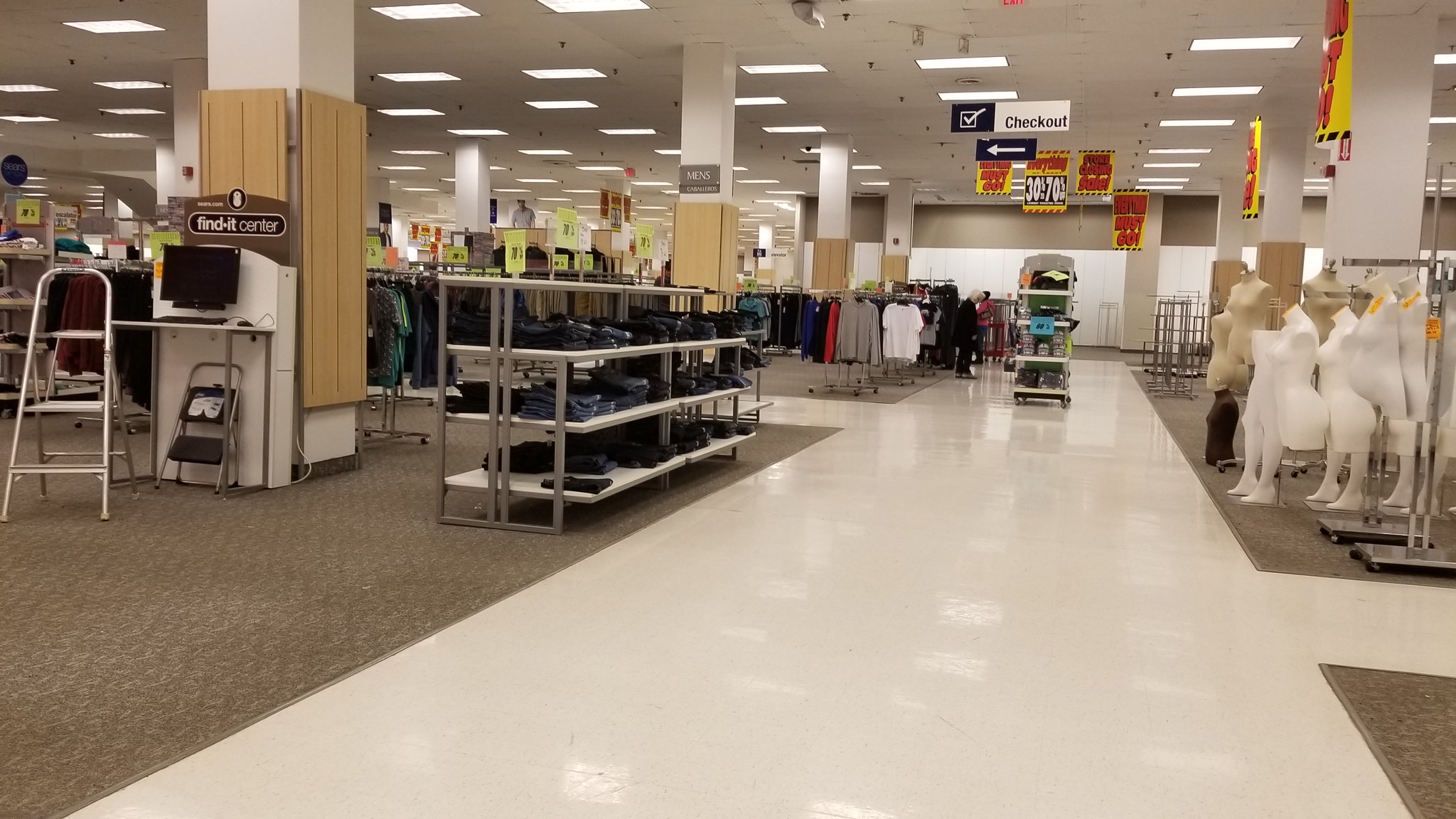The image depicts a department store in the midst of closing down, with clear indications of a large-scale clearance sale evidenced by signs advertising discounts ranging from 30% to 70%. The store's once bustling aisles are now sparsely populated, lending an air of desolation. A large sign indicating the checkout area is prominently visible at the top of the image. On the left side, there are two step stools of different sizes, a larger one and a smaller one, suggesting employees have been using them for packing or reorganizing. The front section of the store is completely empty, mirroring the right side, which features only bare mannequins in a stark, vacant setting. Some scattered clothing items still linger on the remaining racks, mostly concentrated towards the back and the left side of the store. The glossy white floor tiles guide the viewer’s eye towards the back, where a lone figure, possibly a shopper or an employee, is seen, making it hard to discern their role in the scene. The image captures a poignant moment of transition, with the last remnants of merchandise awaiting buyers amid the store’s impending closure.